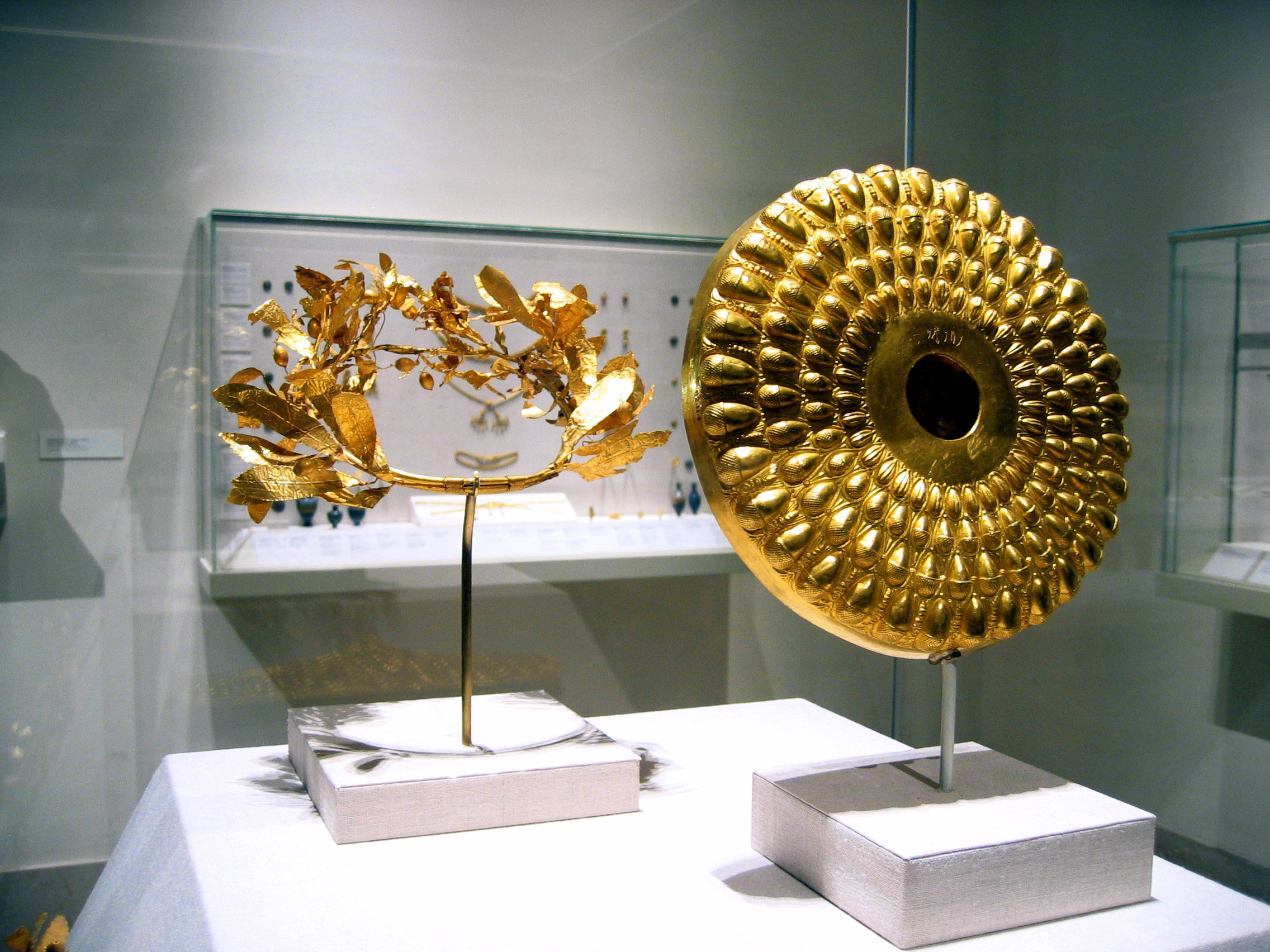This image captures a meticulous artistic display within a gallery setting. Dominating the foreground is an expansive white table, which extends prominently across much of the image. The pristine white walls typical of gallery spaces form a minimalistic backdrop, subtly emphasizing the art pieces. Beyond the table, a glass cabinet adds depth to the composition. Encased in a protective glass case, evident from its barely visible edges and faint reflections, two intriguing objects command attention.

The object on the left is an elegant white box, from which a slender gold stem emerges, culminating in an exquisitely crafted gold wreath. The wreath is reminiscent of those worn in ancient times, designed to be delicately placed in one's hair. Contrasting yet complementing it, the right side of the display features a striking gold disc adorned with intricate embellishments that resemble droplets of water. This disc also floats above a sleek white cardboard box, its ornate details enhancing the display's overall grandeur. Both pieces highlight a blend of classical inspiration and contemporary presentation, drawing viewers into their finely curated details.